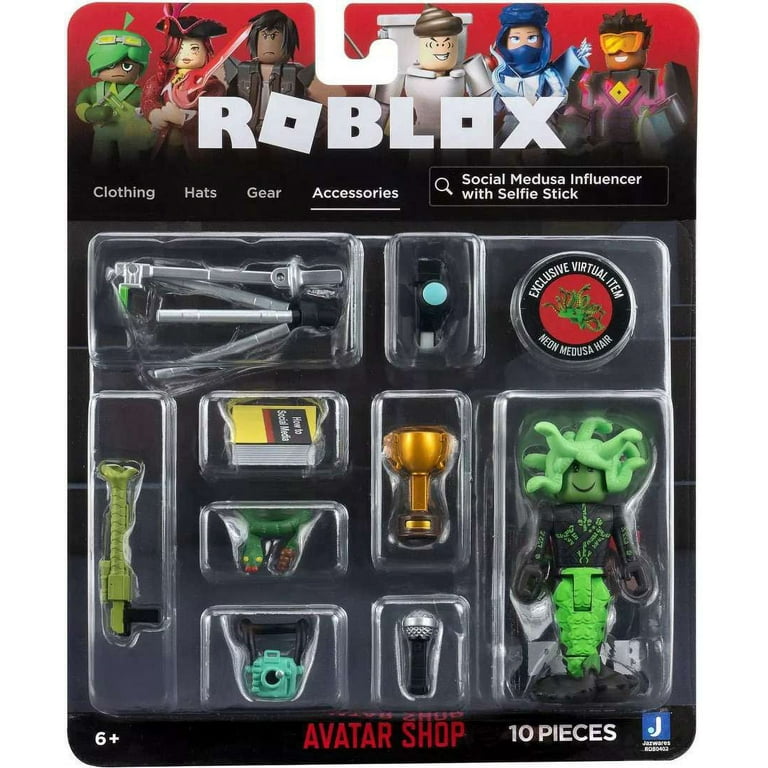This detailed photograph showcases a Roblox toy package designed for retail display, with an L-shaped hook for easy shelving. The package prominently features the word "Roblox" in large, white font at the top, surrounded by various colorful Roblox characters. Labelled as "Social Medusa Influencer with Selfie Stick," the contents target accessories, highlighting items such as clothing, hats, gear, and accessories, with "accessories" notably underlined.

Intended for children aged 6 and up, the package contains a total of ten pieces, emphasized at the bottom right corner next to the text "Avatar Shop." Inside the package, you can find several small plastic items, including the green Medusa-themed influencer character resembling Lego figures, and additional accessories such as a silver selfie stick, blue camera, microphone, trophy, snake, book, tripod, and an exclusive virtual item for the Roblox game, the "Neon Medusa Hair." The package also hints at the vibrant, playful essence of the toy figures and their various accompanying gadgets and gizmos.